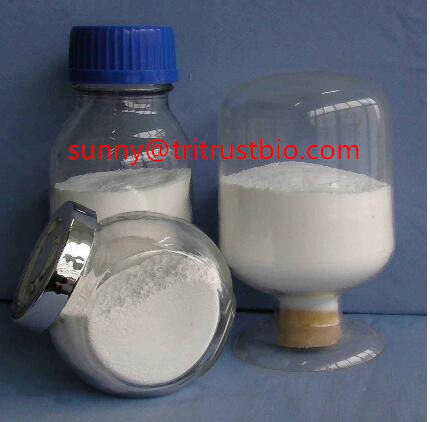The photograph features three containers of white powder arranged horizontally on a blue surface against a blue backdrop that exhibits slight shading due to shadows. The container in the upper left is a mostly cylindrical plastic bottle with a blue, vertically-ridged twist cap that narrows slightly toward the top. This bottle is approximately two-thirds full. Directly in front of it lies a glass jar on its side, with an oval face and a short round silver cap, also around two-thirds full. To the right of these, an upside-down bottle with a wooden cork stands, showing it to be nearly half full. Across the middle of the image, in red lowercase letters, is the email address "sunny@tritrustbio.com," suggesting a connection to a company possibly dealing with botanical or chemical products. The background is a light blue fabric, reminiscent of a couch cushion, with visible seams adding texture and depth to the scene.